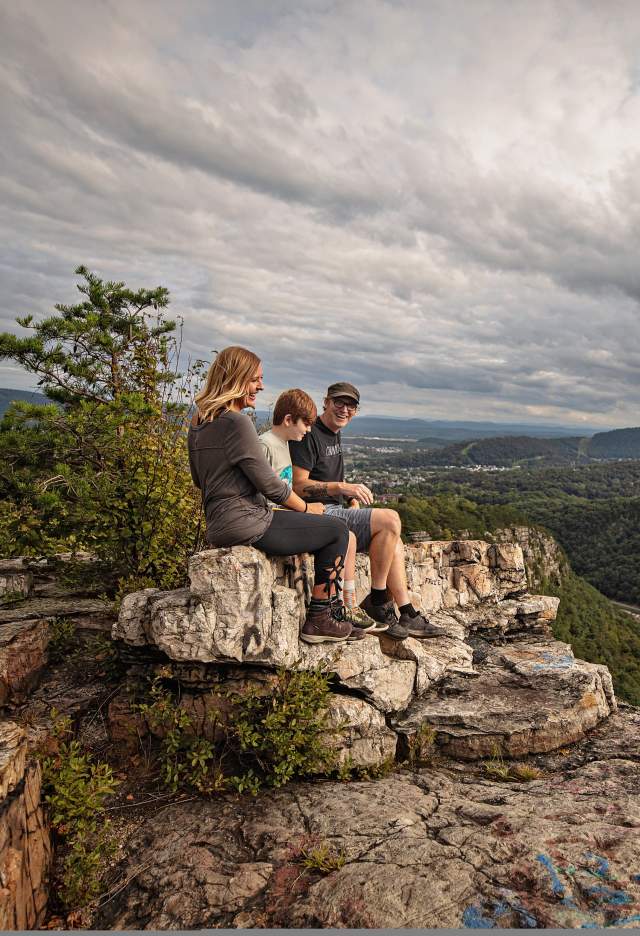This vibrant, portrait-mode photo captures a joyful family of three—presumably a mother, father, and their preteen son—relishing a hiking trip atop a rocky outcrop on a mountain. In the foreground, the blonde mother, clad in gray leggings, a gray shirt, and hiking boots, beams with laughter and smiles warmly. Beside her sits their red-haired son, donned in shorts and a light gray or white t-shirt with a turquoise design. He also mirrors the family’s happiness. To the far side, the father, distinguished by his cap, glasses, black t-shirt, gray shorts, and tattooed arm, shares a laugh while gazing at the mother. 

They are perched on a light tan and gray rock ledge, surrounded by stunted trees and small shrubs. Right below them, some small blue flowers add a pop of color to the rocky setting. Stretched out behind them is a stunning vista of a broad valley dotted with little houses and further encompassed by low hills and distant mountains. The sky above is overcast with gray and white clouds, wrapping the scene in a serene, natural atmosphere. Although they are sitting high on a cliff or bluff, the family’s close connection and shared joy dominate the image, making it a heartwarming snapshot of their outdoor adventure.